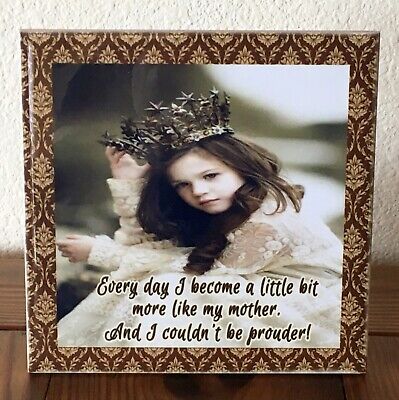This image is a photograph of a framed photograph, captured in a rich brown and gold frame with an intricate, regal design. The frame is resting on what seems to be a wooden surface, placed against a white spackled wall. Inside the frame, a young Caucasian girl is depicted sitting down, gazing pensively to her left. She touches an ornate metal crown adorned with pointy stars. She has long, straight brown hair, fair skin, and brown eyes. Clad in a white lace dress with floral patterns, the girl exudes an air of elegance and innocence. At the bottom of the photograph in a cursive font is the heartfelt text: "Every day I become a little more like my mother, and I couldn't be prouder."